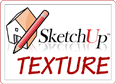This image offers a detailed close-up view of a black and white fabric swatch, featuring a checkered or herringbone pattern. Dominating the frame, the intricate woven texture is accentuated by a watermark across its center, though it is illegible. At the bottom of the image, clear text reads "www.SketchUpTextureClub.com" alongside "free download." In the bottom right corner, there is an inset image depicting a solid and heavy-looking upholstered chair, also adorned with the same black and white pattern. This chair, which has two armrests and short, stout black legs, visually emphasizes the fabric's application in furniture design, making it a likely sample to showcase this particular fabric.